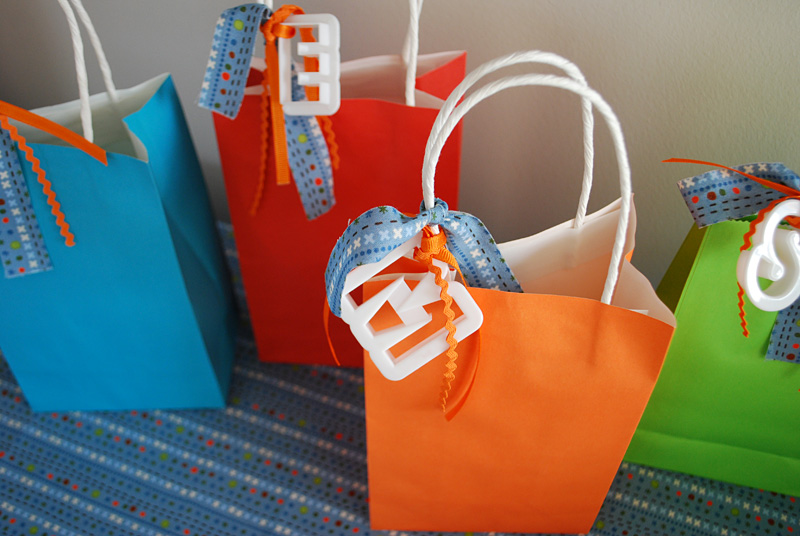The image is a realistic photograph displaying a rectangular composition, wider than it is tall. The setting features a blue, striped, older-looking carpet laid under a cream-colored or light off-white wall. On the carpet, there are four colorful paper gift bags, each with white string handles. Arranged from left to right, the bags are blue, red, orange, and green. The orange and green bags are slightly positioned in the forefront, adding depth to the arrangement. The bags are adorned with both orange and blue ribbons, although the ribbon on the green bag on the right appears almost red. Each ribbon is detailed with red, orange, green, yellow, and blue dots. The mismatched yet coordinated ribbons suggest these gift bags may be parting gifts for a party. The consistent ribbon designs and the structured placement of the bags create an organized yet vibrant visual display against the patterned blue carpet.